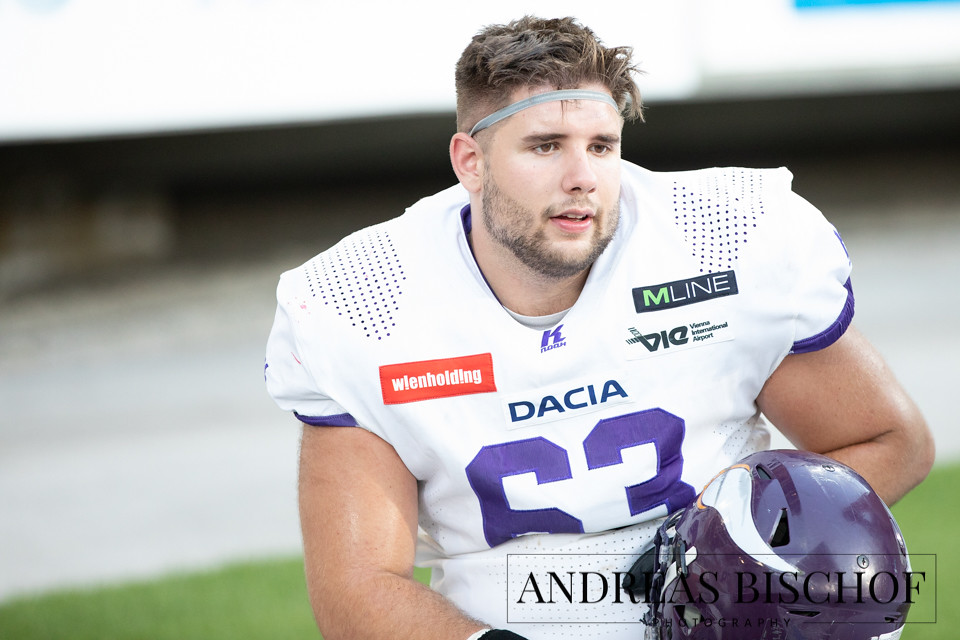This is a posed, full-color outdoor photograph of a young male football player, presumably belonging to the Minnesota Vikings given his white uniform with a purple number 63 and a purple helmet adorned with white horns extending from the front to the back. The athlete is positioned on a blurry field, suggesting greenery in the background. He features a rugged appearance with short brown hair shaved close on the sides and longer on top, held back by a small gray or blue headband. A bit of a week-old beard adds to his rugged look. His fair skin and brown eyes convey a slightly tired expression as he kneels, holding the purple helmet, with only the upper half of his body visible. His large arms hint at a solid build. The uniform bears several sponsor logos, including "Dacia," "Wienholding," and "VIE M-Line," indicative of commercial affiliations. The image credits go to Andreas Bischoff, whose name is superimposed in black letters toward the bottom right of the image.